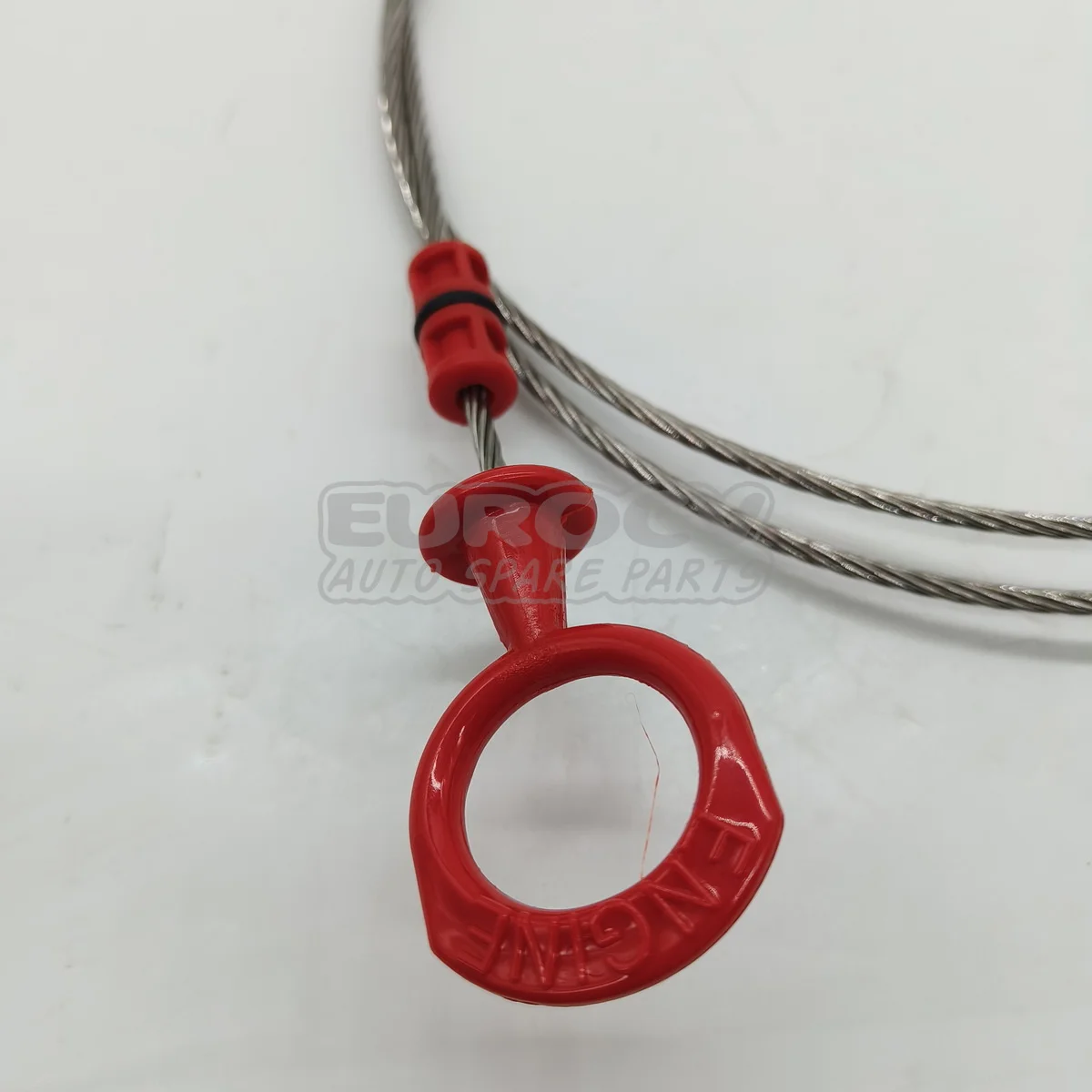This detailed close-up image shows a braided metal cord, likely an automobile part, with a watermark in the center reading "Euro C1 Auto Spare Parts." The cord has a metallic, double rope-like structure, appearing shiny and silver. Extending from the cord is a distinct red pull handle, composed of red plastic nuts connected by thin black washers. The handle terminates in a round, red plastic cap with the word "ENGINE" clearly written in capital letters. The handle is designed to be pulled, similar to a lawnmower pull cord, with a hole for a finger to grip. The background is plain white, casting a top-down shadow of the cord.